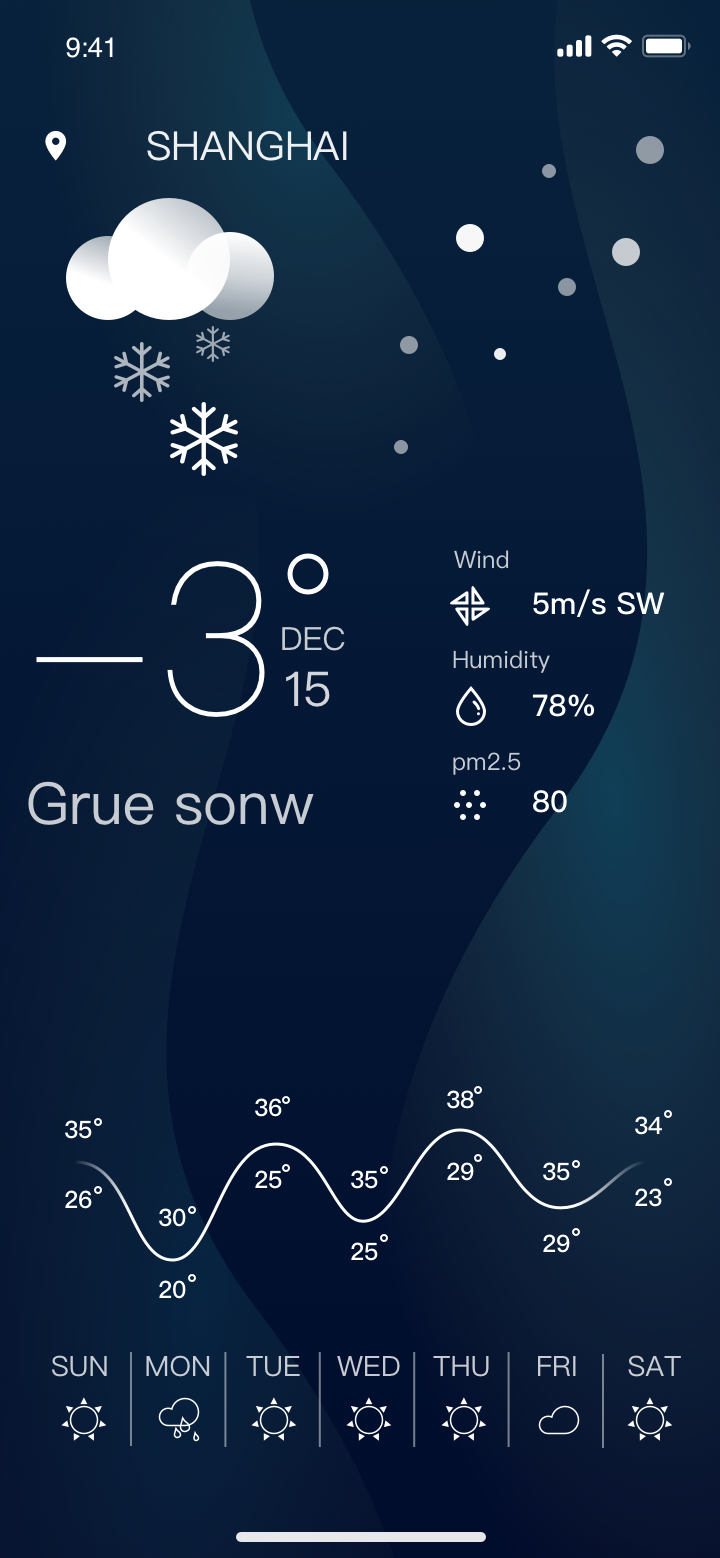A detailed caption for this image could be:

"This screenshot appears to be taken from a mobile phone, displaying a weather app with a dark blue background featuring vertical swirls running from the top to the bottom of the screen. In the status bar at the top, the time is shown as '9:41' on the left, while the right side displays icons for battery, cell signal, and Wi-Fi signal strength. Beneath the status bar, a location icon next to the text 'SHANGHAI' indicates the city, written in all capital letters and white text.

Below the location, there are three round circles, with the middle one being the largest, accompanied by animated snowflakes descending. To the right, bubbles can be seen. The temperature is displayed as '-3°C,' followed by the date 'December 15,' wind speed '5 mph,' and humidity level '73%.' Additionally, the air quality index is noted as 'PM 2.5: 80,' and a cryptic string 'GRUE NONW' appears.

Further down the image, there's a graph resembling a wavy line, featuring several peaks and troughs indicating varying data points: '35, 26, 30, 20, 36, 25, 25, 25, 38, 29, 35, 29, 34, 24.' At the very bottom, the days of the week are listed from 'Sunday' to 'Saturday.'"